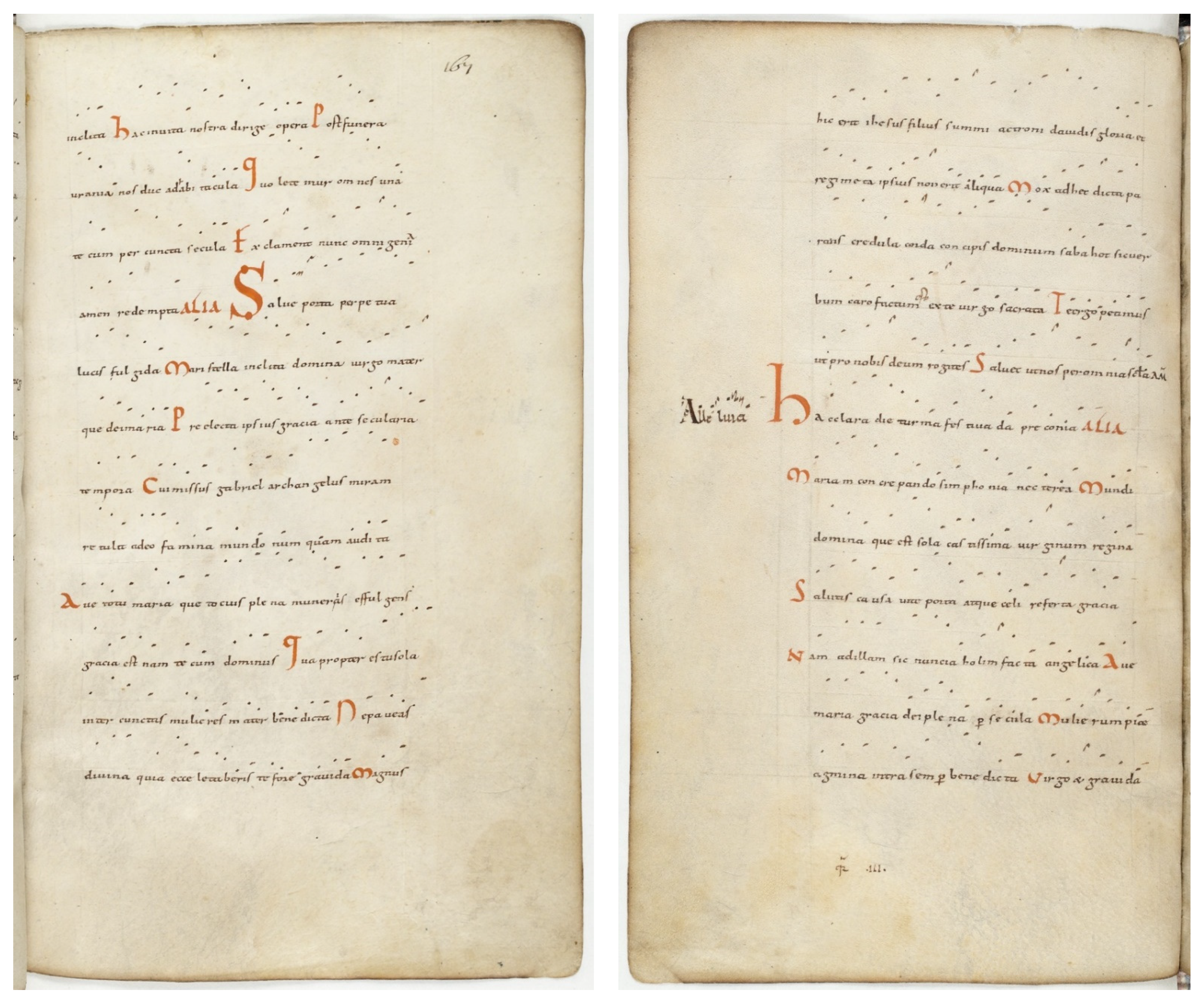The image showcases two color photographs of different pages from the same book. Both pages appear worn and aged, suggesting the book is quite old. Each photograph displays a section from the opposite side of the book, with the left photograph featuring the right page and the right photograph featuring the left page. The text on these pages is primarily printed in black ink, but prominently features ornate and larger letters, such as several "M"s and an "H," highlighted in red ink, which stand out against the rest of the text. The language and script suggest that the text is an ancient or religious document, not in modern English. The photograph is clear and well-lit, making the details of the decorations and text easily visible despite the age-worn appearance of the pages.